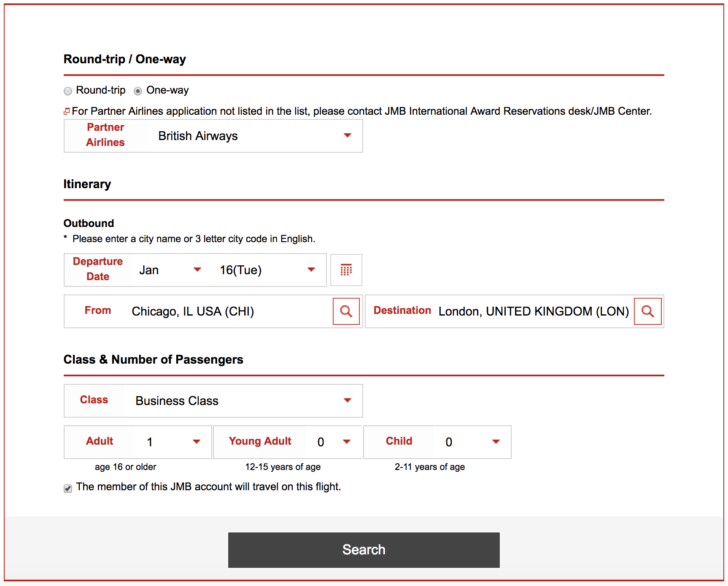The image showcases an airline booking form divided into three distinct sections, each with pertinent travel information neatly categorized for user input. All text is in black, while key elements such as section titles and drop-down labels are highlighted in red and underlined, making the interface visually intuitive.

1. **Travel Type**:
   - **Title**: "Round Trip or One Way"
   - **Details**: Options provided are "Round Trip" and "One Way." In this instance, "One Way" is selected.
   - **Notification**: A note advises that for partner airlines not listed, users should contact the JNP International Award Reservation Desk or the JNP Centre.
   - **Dropdown Menu**: A dropdown at the bottom states "British Airways Partner Airlines," with "Partner Airlines" in red and "British Airways" in black.

2. **Travel Itinerary (Eternal Rally)**:
   - **Title**: "Eternal Rally"
   - **Outbound Information**:
     - Users are prompted to enter a city name or three-letter city code in English.
     - A dropdown menu indicates the departure date, "January 16th, Tuesday," with "departure date" and "from" highlighted in red.
     - Departure details: "From Chicago, IL, USA (CHI)"
     - Destination details: "To London, United Kingdom (LON)"
     - Both the search bars for city codes are visually marked in red for ease of use.

3. **Class and Number of Passengers**:
   - **Title**: "Class and Number of Passengers"
   - **Class Selection**: The class is set to "Business Class."
   - **Passenger Details**:
     - Adults: 1
     - Young Adults (12-15 years): 0
     - Children (2-11 years): 0
     - Infants (under 2 years): 0
   - **Member Verification**: A checkbox confirms that the member of the JNP account will travel on this flight.

At the bottom of the form is a dark grey search button. The image suggests an informative and user-friendly interface designed for efficient flight reservations.